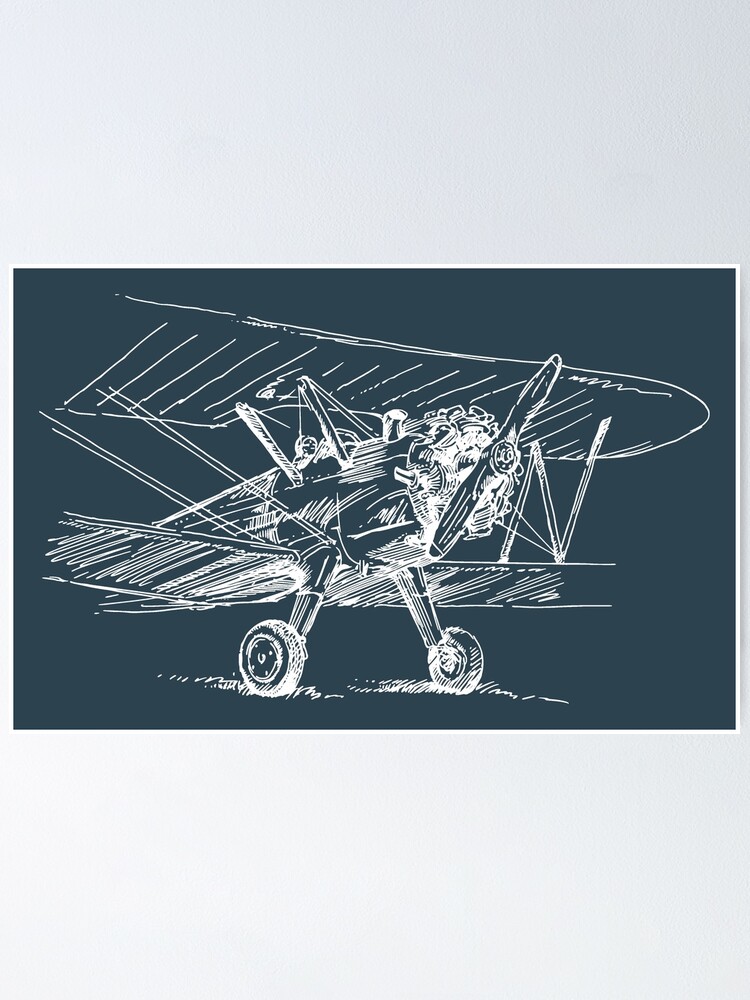This image appears to be a detailed scratchboard-style illustration, set against a dark blue-green, solid background. The technique used involves white lines on the dark background, reminiscent of early aviation art. The subject is an early model biplane, identifiable by its two sets of wings—one above and one below the plane's main body. The structure includes vertical supports and wires that connect and tether the wings. At the front, there is a propeller with two blades positioned vertically. The plane’s body is designed like a long capsule, suggesting the rudimentary shapes of early aircraft designs. Two wheels are visible, indicating that the aircraft is grounded on grass. There also seems to be the faint outline of a possible pilot in the cockpit, emphasizing its historic nature. Overall, this illustration captures the essence of one of the first airplanes from the pioneering days of aviation.